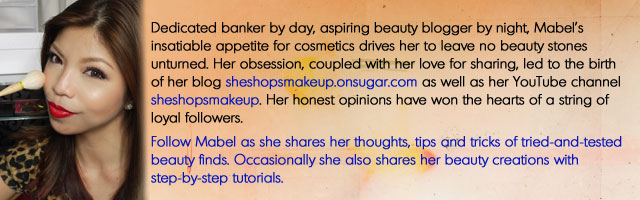The image depicts an Asian woman standing in a kitchen on the left side, her brown hair framing her face as she applies blush with a makeup brush. She is wearing an animal print shirt and has expertly applied eyeliner, mascara, and red lipstick. The woman is introduced as Mabel, a dedicated banker by day and an aspiring beauty blogger by night. The accompanying text highlights her insatiable appetite for cosmetics and her passion for sharing beauty tips, which led to the creation of her blog, SheShopsMakeup.onsugar.com, and her YouTube channel, SheShopsMakeup. Known for her honest opinions, Mabel has garnered a loyal following. She regularly shares her thoughts, tips, and tricks on tried and tested beauty products and occasionally posts step-by-step tutorials of her beauty creations. The text is set against a peach-colored background.